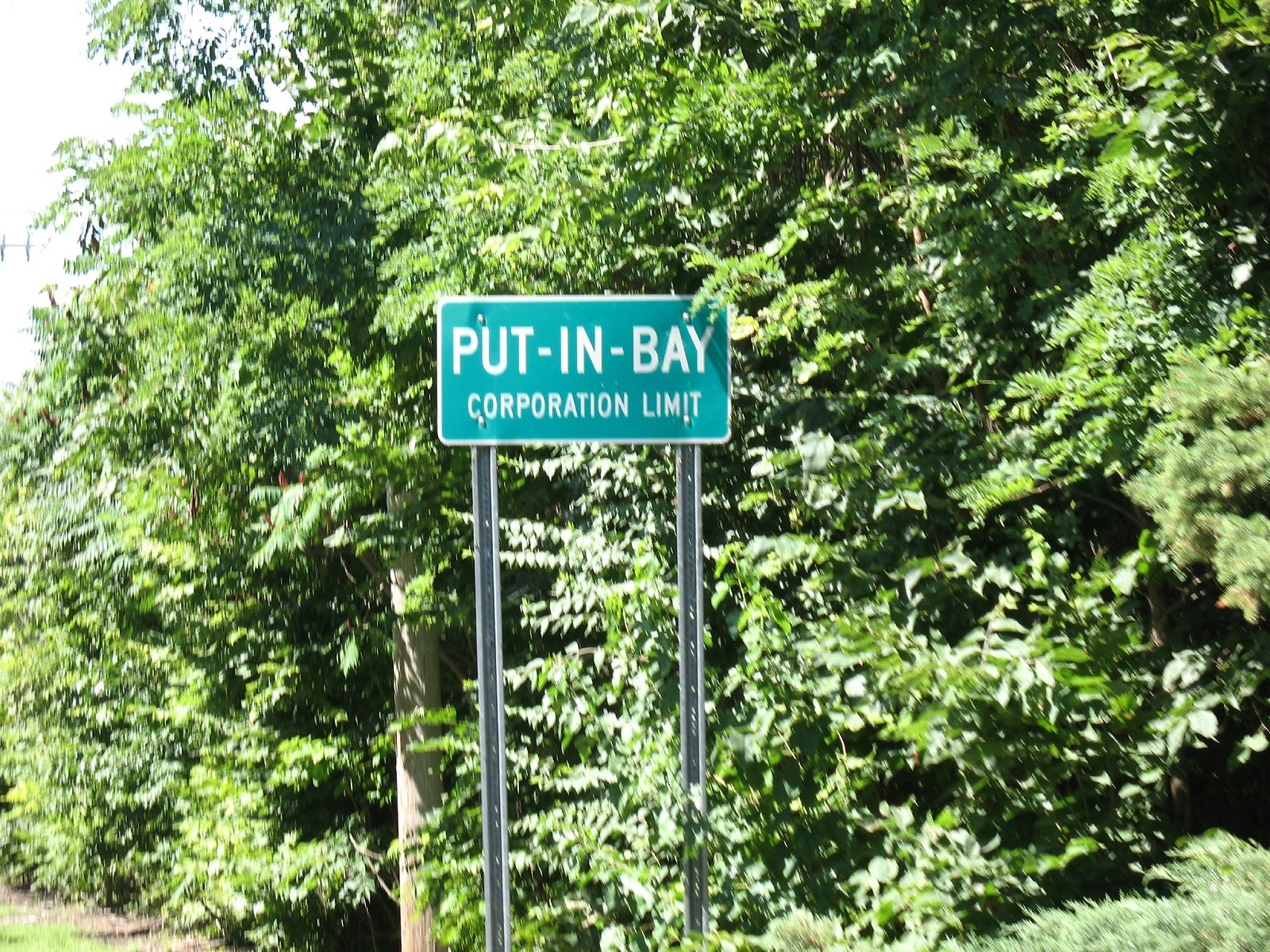This image features a prominent roadside sign supported by two long, silver metal signposts. The rectangular sign is green with a white border and bold white lettering that reads "Put-In-Bay Corporation Limit," with dashes between each word and "Put-In-Bay" in larger letters. The backdrop consists of lush, green foliage, primarily large, fully-leaved trees, and a visible tree trunk, creating a predominantly green landscape. Above the dense trees, a light grey, overcast sky can be seen, adding a soft contrast to the vibrant greenery below. The bottom part of the image cuts off just before reaching the ground level, suggesting the sign is situated at a height. Overall, the setting appears to be an outdoor area embellished with rich greenery and a muted sky.